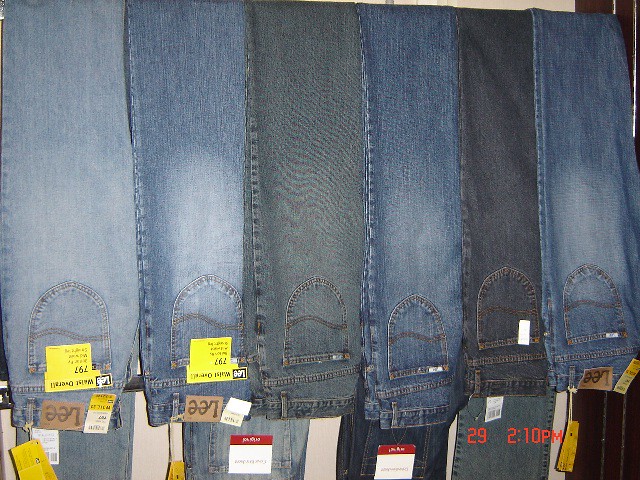The image depicts a market stall or a section within a department store showcasing denim jeans. There are six pairs of Leigh jeans prominently displayed, draped over a pole for display purposes. These jeans, identifiable by their tags, are organized by color from light to dark shades, including a light to medium tone, various darker blues, and a pair with a grayish base. Behind these are five more pairs of jeans. All pairs are tagged, with the signature yellow tags and sale price tags hanging conspicuously. The photograph appears amateurish, marked by an old-school digital photo time stamp. While the focus remains on the diverse shades of blue jeans, there is a slight glimpse of creamy wool fabric in the background.